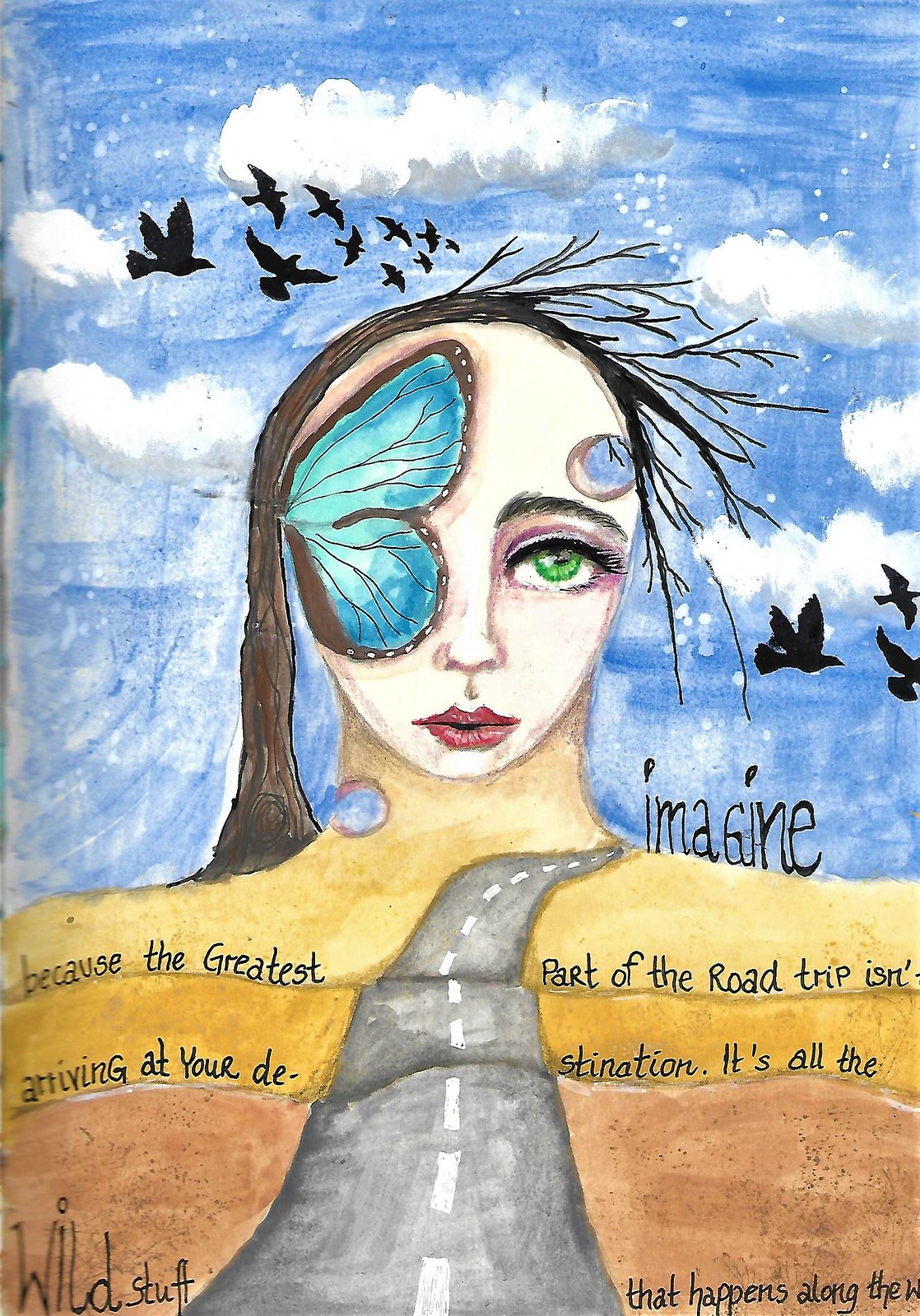The painting is an abstract depiction featuring a nuanced convergence of nature and human elements. In the far background, a blue sky rendered with crayons or watercolors is filled with various white and gray clouds, and multiple outlines of birds flying through the sky. Central to the image is a woman's head; her left eye is obscured by the delicate, blue wing of a butterfly, while her right eye is a striking green, looking upwards. Her lips are painted a vibrant red, and her nose is clearly defined. The left side of her hair is brown, contrasting with the right side, which is composed of tree trunks and twigs extending outward. There's a conspicuous hole on the right side of her forehead, through which the sky is visible. Beneath this, her neck transitions into a landscape, depicting a dirt road flanked by textured ground that flows seamlessly up to her head. The word "Imagine" is inscribed in black letters across the blue sky, and an extended quote above her neck area reads, "because the greatest part of the road trip isn't arriving at your destination. It's all wild stuff that happens along the way." The chest area gradients from yellow to brown, and features additional text. This imaginative scene melds natural and surreal elements, inviting viewers to explore its myriad intricacies.